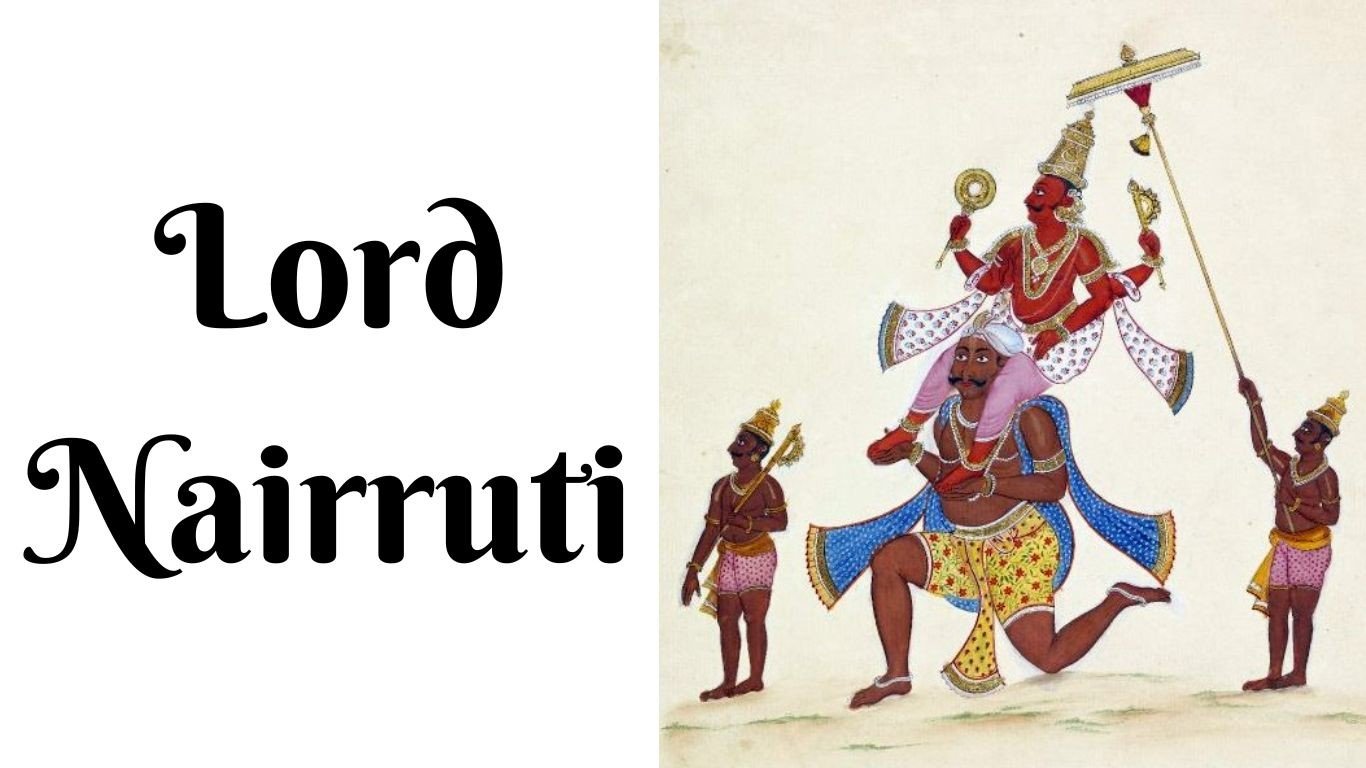The image is divided into two distinct sections. On the left, against a stark white background, the text "Lorde, Nairuti," spelled N-A-I-R-R-U-T-I, is prominently displayed in large black letters. The right side reveals a detailed illustration set against a cream backdrop. Central to the scene are four Indian characters depicted on a dirt ground peppered with small grass patches. In the middle, a heavyset man with red skin, kneeling on one knee while his other foot is firmly planted, wears yellow shorts with red designs, sandals, and a blue robe. He is supporting a slightly smaller man on his shoulders. This smaller individual, adorned in a white robe, pink pants, and a crown, wields two golden scepters in his hands. Flanking them are two even smaller men, each wearing pink shorts with red designs and small crowns similar to the one worn by the figure on the shoulders. The man on the left merely stands in his shorts and jewelry, while the man on the right holds an ornate umbrella on a long pole, seemingly providing shade or a ceremonial cover.